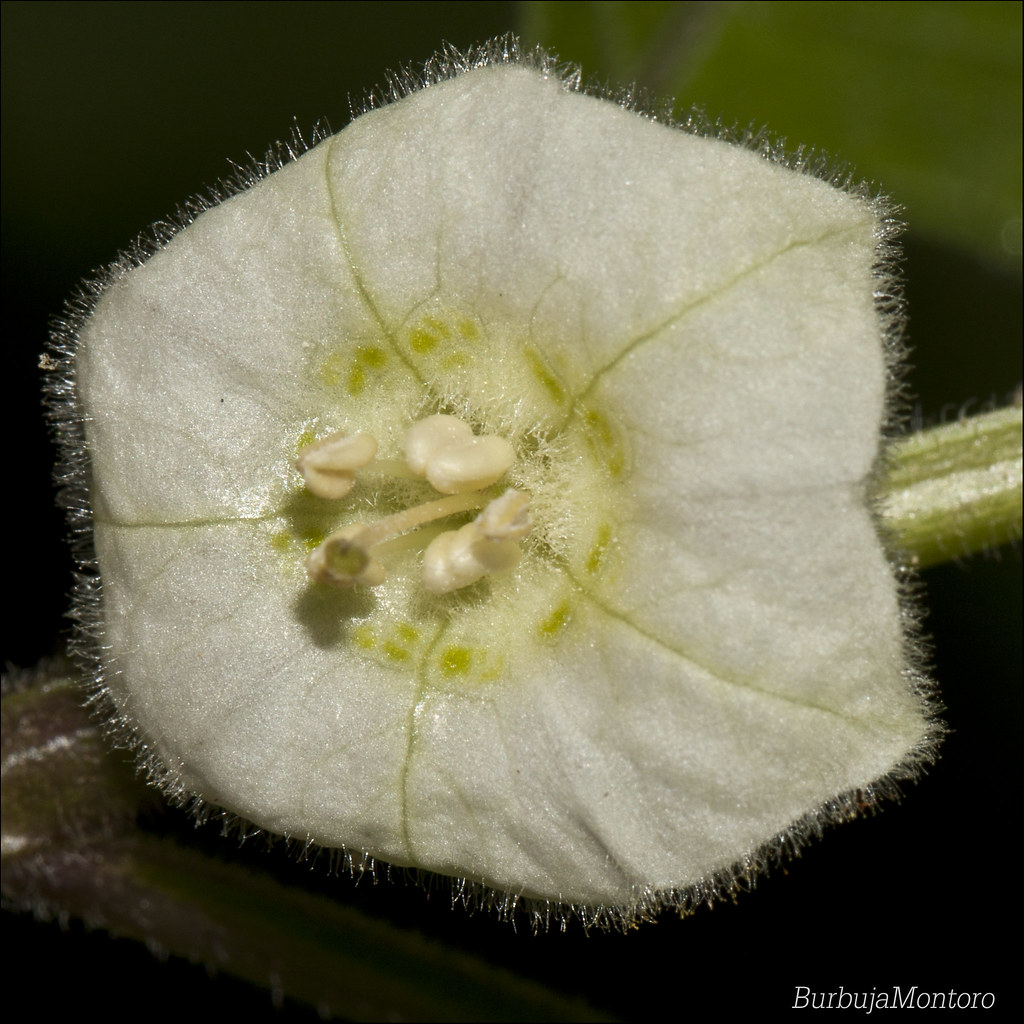The photo, taken in a dimly lit room or at night, features a striking, fuzzy white flower with a unique star-shaped design, resembling a zucchini flower. The flower consists of a single petal divided into five distinct upside-down triangles by green veins. The center of the flower has a greenish hue, adorned with delicate white pollen structures protruding slightly. The flower has a hairy or fuzzy appearance, with shiny hairs accentuating its texture. In the background, a green stem can be discerned amidst a blurred backdrop. Notably, the bottom right corner of the image is marked with the name Barbara Montoro, possibly the photographer.